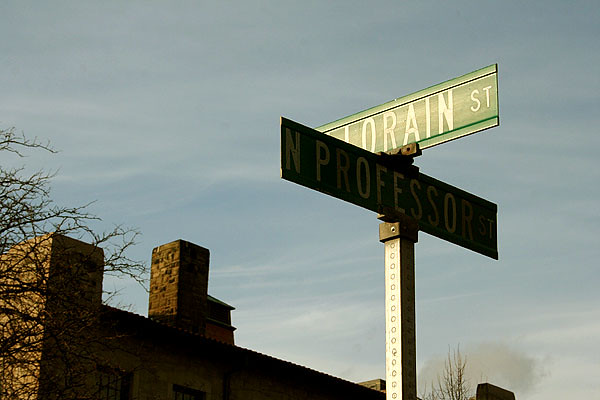The image captures an outdoor scene featuring a street sign at the intersection of North Professor Street and Jordan Street. The signs are green with white lettering, with Jordan Street more illuminated compared to the darker North Professor Street sign. In the background, a light blue sky is adorned with patches of gray and white clouds, and gray, wispy formations that could be smoke. To the left of the street signs, barren tree branches add a stark contrast as they stretch out without leaves. A brick building, possibly with a chimney, emerges near the base of the tree and extends just behind the street sign, further illustrating the urban setting.